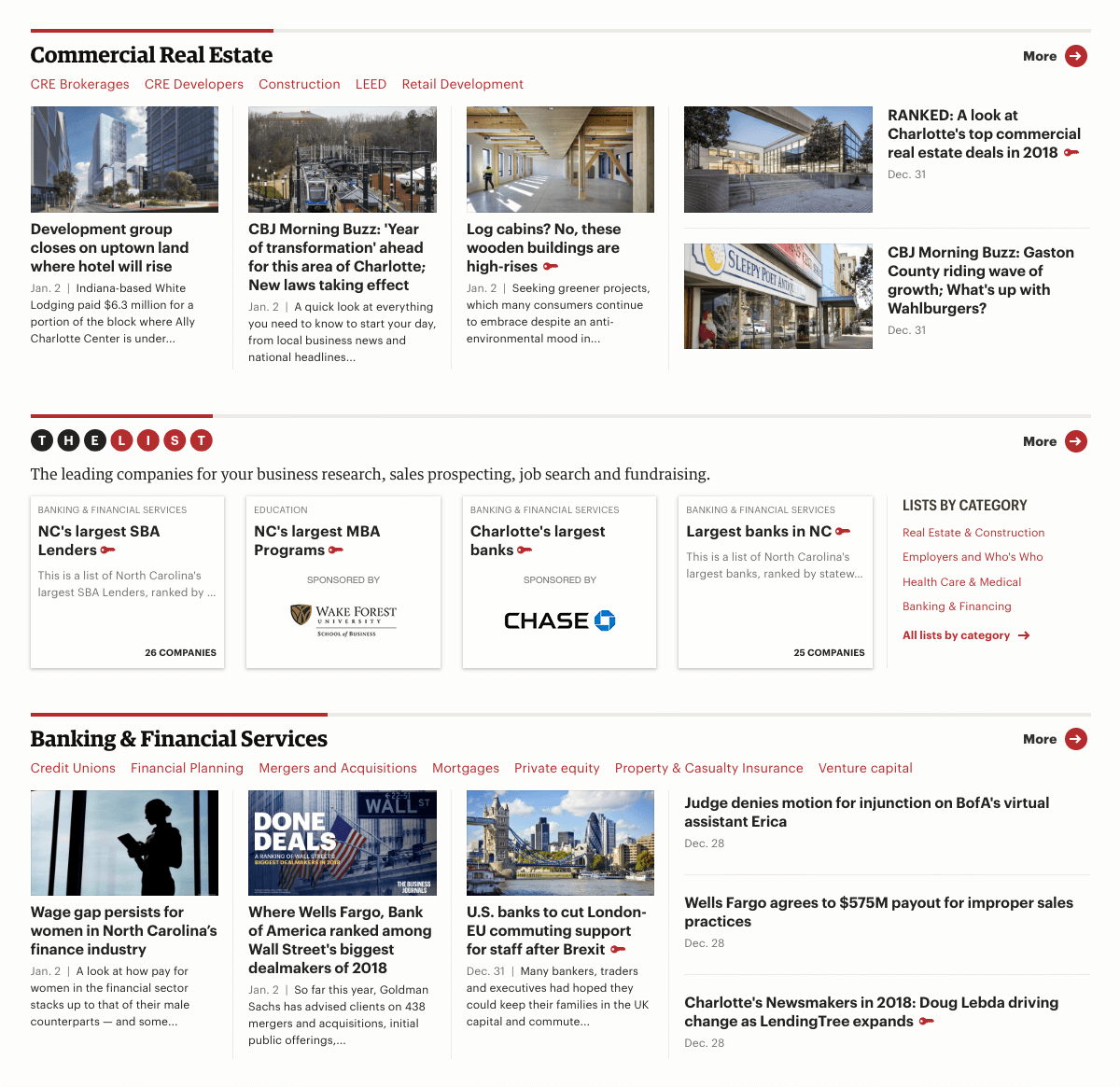Homepage Screenshot: A Comprehensive Financial and Real Estate News Website

The homepage presents a dual-focused design, catering to both commercial real estate and banking & financial services interests. Positioned at the top is a sleek navigation bar, though the site name remains elusive. Below, the page divides into two primary sections filled with dynamic content.

On the left, under the "Commercial Real Estate" banner, users can explore a variety of articles through a horizontally scrollable interface. Prominent headlines include:

- "Development Group Closes on Uptown Land Where Hotel Will Rise"
- "Log Cabins: None of These Wooden Buildings Are High Rises"

A "More" button invites users to delve deeper into a repository of related content.

To the right, the "Banking and Financial Services" section mirrors the layout, offering notable pieces such as:

- "Wage Gap Persists for Women in North Carolina's Finance Industry"
- "US Banks to Cut Lending, EU Commuting Support for Staff After Brexit"

This layout lends the site a comprehensive, one-stop-shop feel for financial news enthusiasts, likely operating as an aggregator consolidating varied industry updates in one streamlined location.